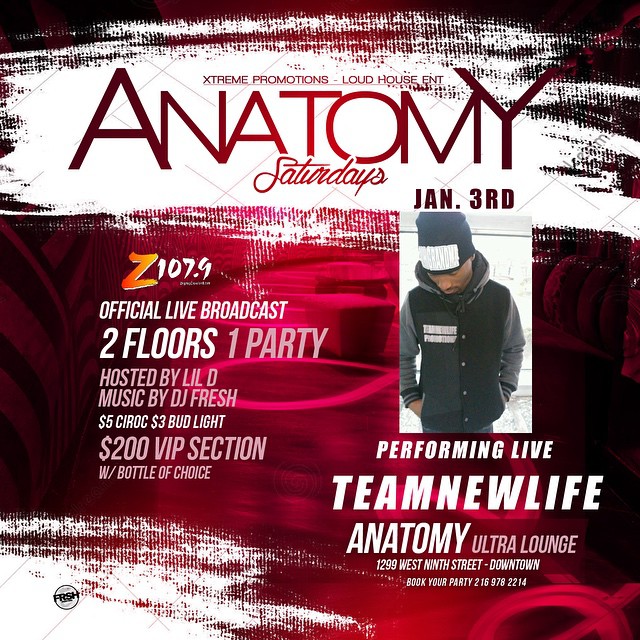The image is a detailed advertisement flyer for an event. The background features a gradient of maroon and rosy pinkish-red hues, with the top portion whitewashed for emphasis. Prominently, the top of the flyer showcases the text "Extreme Promotions Loud House ENT" followed by "ANATOMY" in capital letters, with "Saturdays" elegantly inscribed in cursive underneath. Below this, in impact font, it reads "January 3rd."

On the right side of the flyer, there's a photograph of an African-American male with brown skin wearing a black jacket with gray sleeves and a black beanie hat, which has white text on it. The details of the jacket's text are not readable. To the left of the image, the text announces, "Z107.9 official live broadcast, two floors, one party" and mentions that the event is "hosted by Lil D, music by DJ Fresh."

Additionally, the flyer lists various promotions: "$5 CIROC," "$3 Bud Light," and a "$200 VIP section with a bottle of choice." Beneath the photograph, further details include an announcement for a live performance by "Team New Life" at the "Anatomy Ultra Lounge," located at "1299 West 9th Street downtown." It also encourages party bookings followed by a contact phone number. The overall color scheme blends reddish tones with maroon and white, giving the flyer a vibrant and eye-catching look.